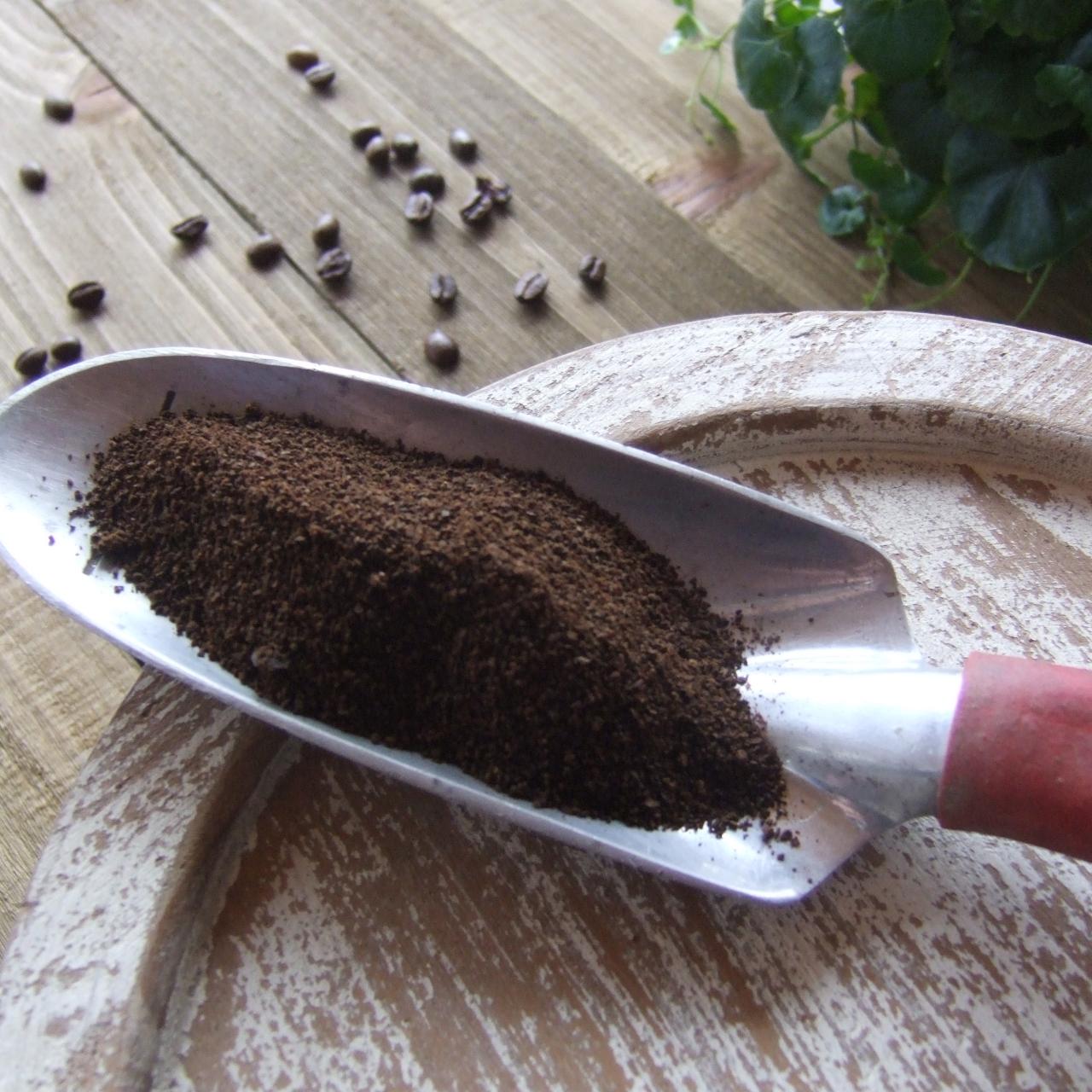A beautifully detailed garden scene captures the essence of rustic charm. Center stage is a garden trowel with a striking red handle and a glistening silver blade, suggesting imminent use in the garden. The trowel rests atop a weathered wooden barrel, adorned with streaks of antique white paint that evoke a sense of timelessness. Adjacent to the trowel sits a scattering of freshly ground coffee beans on a rich wooden surface, their deep color contrasting with the lighter shades of the barrel. In the upper right-hand corner, a delicate ivy plant adds a touch of greenery, further enhancing the vintage atmosphere of the setting. This image evokes a sense of homeliness and nostalgia, blending gardening and daily rituals seamlessly.